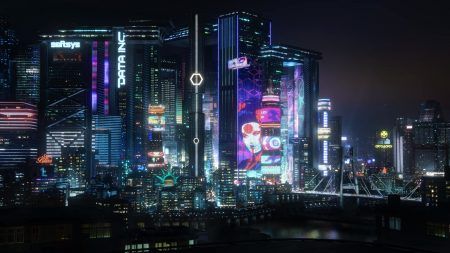This image depicts a sprawling urban skyline at nighttime, dominated by towering, colorful skyscrapers bathed in vibrant neon hues of blues, purples, pinks, and yellows. The majority of the tall, illuminated skyscrapers cluster towards the left and middle sections of the cityscape, progressively giving way to shorter buildings and a visible bridge that spans from the right to the middle of the image. A striking element is a large face painted on one building, reminiscent of traditional Japanese makeup, suggesting an Oriental influence, possibly Tokyo. The scene is rich with digital and neon signage, including a prominent "Data Incorporated" sign atop a skyscraper, adding a technological ambiance to the city. The nighttime sky transitions from dark black on the left to a slightly lit dark brown on the right, further contrasting with the vibrant city lights. At the bottom, towards the right, there is a dark expanse resembling a body of water, adding depth to this mesmerizing and technologically infused skyline.